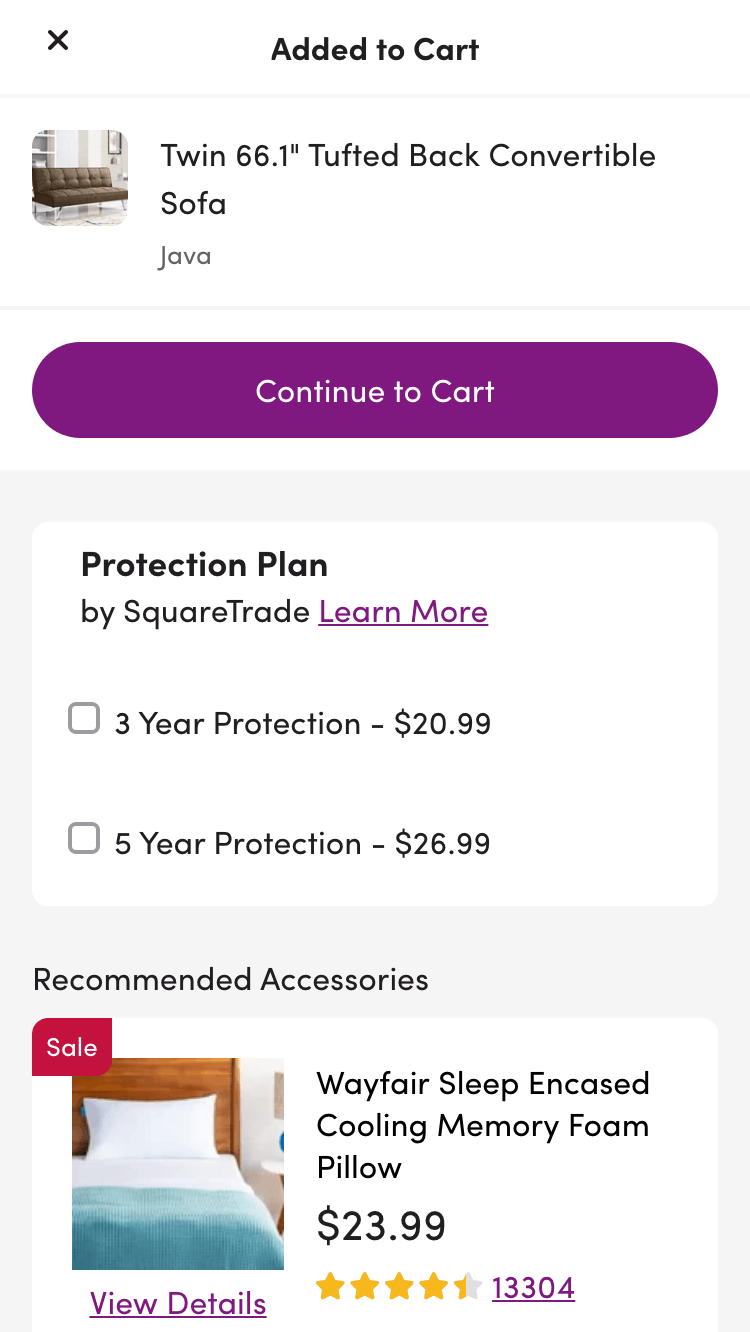The image displays an online shopping screen from Wayfair. At the top, a notification in black reads "Added to Cart," with a black "X" button below it for closing the notification. Below, the product information for a "Twin 66.1 Tufted Back Convertible Sofa" in the color Java is shown, with an option to "Continue to Cart."

Further down, there is an offer for a "Protection Plan by Square Trade" highlighted in purple with a "Learn More" link. The available protection plans are listed as a Three-Year Protection Plan for $20.99 and a Five-Year Protection Plan for $26.99.

Following the protection plan details, there is a "Recommendations" section featuring "Recommended Accessories." The highlighted product is a "Wayfair Sleep Encased Cooling Memory Foam Pillow," marked with a "Sale" tag on the top left. The product image is displayed along with its price of $23.99. The pillow has a rating of four and a half stars based on 13,304 reviews. There is also a purple "View Details" button to click for more information about the pillow.

The image thoroughly details the information for the Wayfair items and the associated options available for purchase and protection.